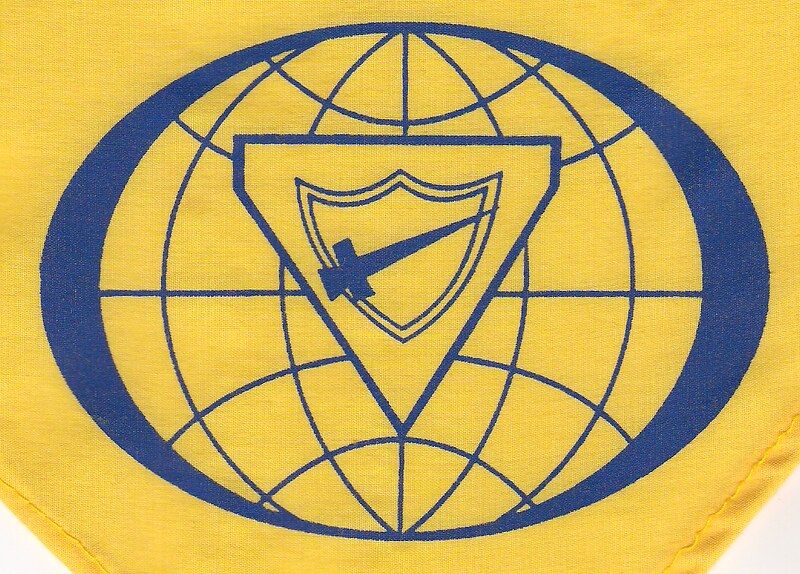This image features a photograph of a yellow cloth that may be a flag, towel, or item of clothing, characterized by intricate stitching at the bottom edges. At the center of the yellow fabric is an elaborate blue design. The design begins with an oval resembling a globe, marked by blue lines that suggest global segments. Overlaying the globe is a simple outlined, upside-down triangle which encloses a similar outlined shield. Diagonally crossing the shield is a solid blue sword or dagger, the only completely filled blue object in the image. This distinctive arrangement creates a layered, symbolic emblem that stands out prominently on the fabric.